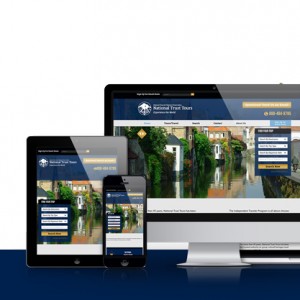In this image set against a minimalist white background, three electronic devices are prominently displayed in realistic photographs. In the upper right, a sleek black monitor with a silver base is showcased. Its screen features a picturesque scene of a canal adorned with distinctly Italian architecture. Neighboring the monitor on the lower left is a modern tablet, displaying the same idyllic canal scene. The tablet's interface includes a menu on the lower left with four white options and one highlighted in yellow, along with a white footer at the bottom of the screen. To the right of the tablet, a black cell phone is positioned. Although the screenshot on the cell phone is somewhat blurry, it unmistakably portrays the same canal scene, featuring reflections of a row of buildings and homes. Additionally, lush greenery lines the left side of the canal, accompanied by a rock wall at the lower right corner of the photo.